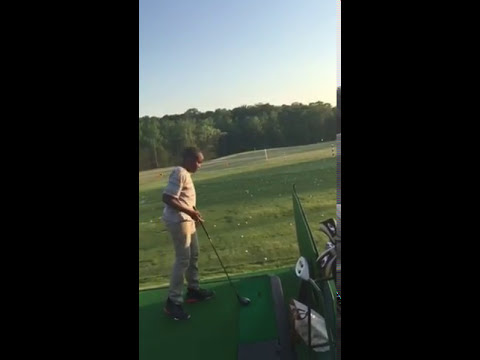The image captures a 13-year-old African American boy practicing golf on a driving range. He is dressed in a tan shirt with brown and yellow stripes, tan pants, and black tennis shoes. Positioned on an AstroTurf green, he holds a golf club and looks down at the ground. To his right is his golf bag filled with clubs. Several flags stand about 150 yards ahead of him, marking different distances, and beyond the driving range stretches a grove of tall trees. The sky above is clear, transitioning to a dusky hue, suggesting the sun is setting, while the overall backdrop includes green grass and multiple shades of green and brown from the trees and foliage. The scene is a square framed photograph, with the boy slightly to the left and the golf equipment to the right.